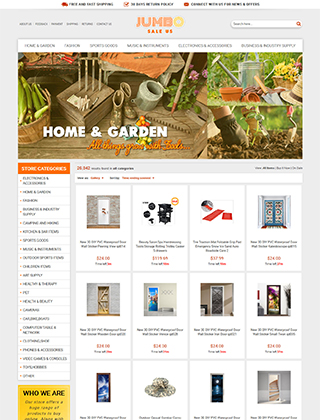The website for Jumbo, an e-retailer specializing in gardening supplies, features a vibrant and welcoming homepage. The company name "Jumbo" is prominently displayed at the top, with "Jumb" in orange and the "O" in yellow, accompanied by a "SALE" banner. The main graphic showcases a picturesque garden scene, replete with a barrel of corn, a pitchfork, a rake, muddy gumboots, a watering can, pot plants, wooden crates, shovels, terracotta pots, and a hand planting in soil. Overlaying this image in bold white text are the words "Home and Garden," while an inspirational orange cursive script reads "All Things Grow with Tools."

On the left-hand side, a sidebar lists the store categories in a long rectangular menu. To the right of this, a grid of windows displays various items currently on sale, offering shoppers a quick view of promotional products. The clean and organized layout invites gardening enthusiasts to explore a variety of sunhats, screen doors, gardening equipment, and advanced watering systems available for purchase.